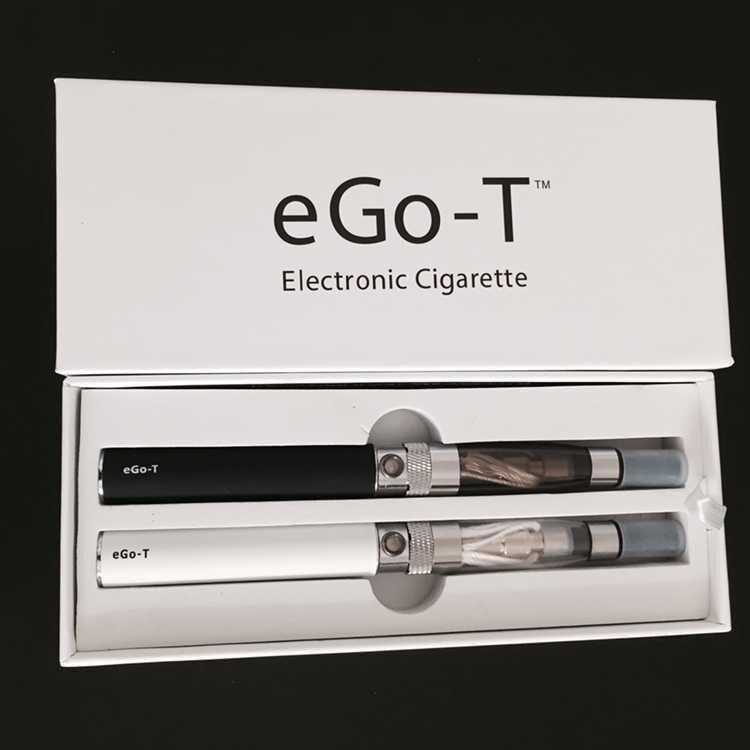The image features a white, rectangular case for an EGO-T electronic cigarette set against a black background. The open case displays its contents, which include two electronic cigarettes—one black and one white—each with metal buttons in the middle and light blue plastic covers on the tips. The top lid of the case prominently displays the trademark "EGO-T" in black text, with "electronic cigarette" written underneath. At the bottom right corner of the image, against the black background, are the words "DHgate.com" and "Atomizer88," suggesting the case's promotional nature.